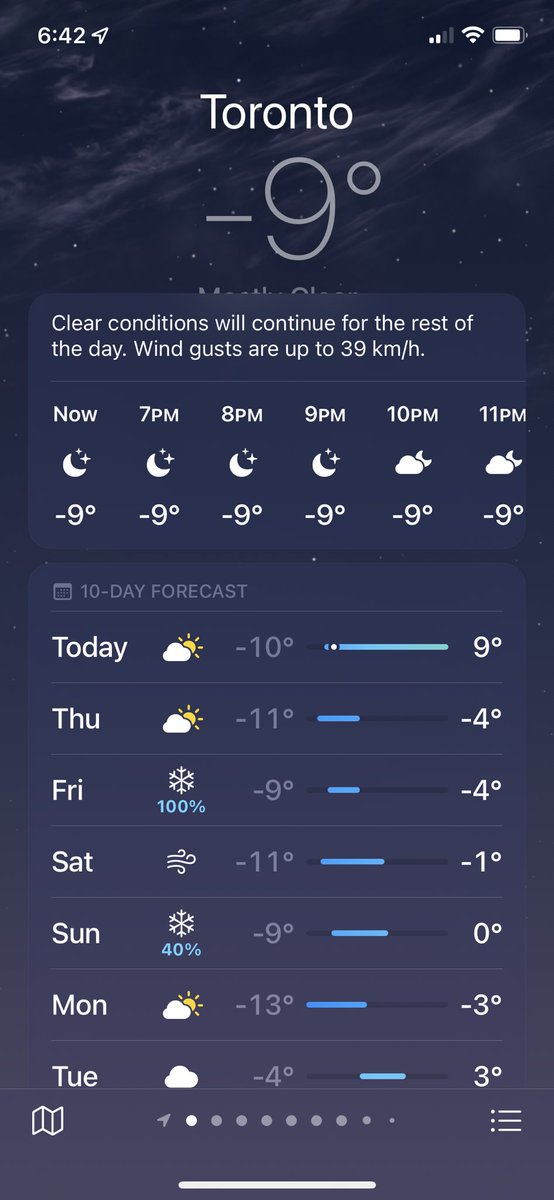An image captured from a smartphone's weather application, displayed in a vertical orientation, showcasing detailed nighttime weather information. The background features a serene night sky with wispy white clouds against a dark navy backdrop, sprinkled with tiny white stars, enhancing the nocturnal atmosphere.

In the upper portion of the screen, the status bar is visible. On the left, the time is shown as 6:42, accompanied by a small location icon. On the right, icons representing signal strength, Wi-Fi connectivity, and battery life are present.

Centered prominently in large white font is the city name "Toronto," with the current temperature of -9 degrees displayed in gray directly below. A darker gray overlay box informs users that "Clear conditions will continue for the rest of the day," with an additional note about wind gusts reaching up to 39 kilometers per hour.

The image further details the weather forecast for the evening hours, providing information for 7 p.m., 8 p.m., 9 p.m., 10 p.m., and 11 p.m. Each hourly forecast includes a small icon, such as the moon or clouds with a moon, alongside the respective temperatures.

Additionally, a "10-day forecast" section is visible, showing a calendar spanning from today to next Tuesday. Each day’s weather includes an icon representing the conditions, the forecasted high and low temperatures, and a bar indicating the range of temperatures.

At the bottom of the screen, a scrollable section allows users to view weather information for different cities, expanding the app's utility for those monitoring multiple locations.